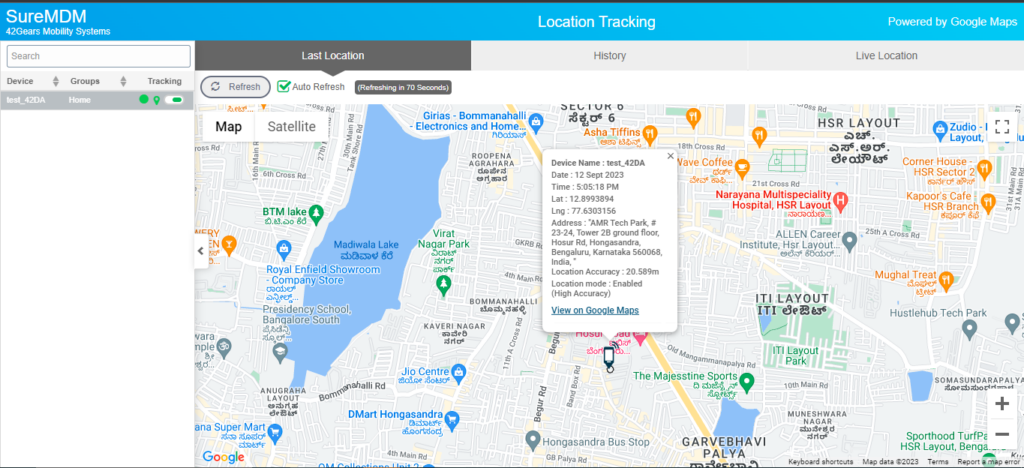This image showcases a location tracking application or website. At the upper left-hand side, the header features the text "SureMDM" in white font, with a capitalized 'S' and 'MDM', while 'ure' is in lowercase. Directly below this, there is a blue bar extending horizontally across the screen. Within this bar, in the middle, it says "Location Tracking" also in white font. Beneath this header section, you can see the main content of the website or app.

On the left side, there is a vertical search section designed for user navigation and queries. To the right of this search section, taking up the majority of the screen's center and right areas, is the main display window, which prominently features a map. This map displays various markings indicative of different locations. Additionally, there is a cell phone icon visible on the map, showing that a mobile device is currently being tracked.